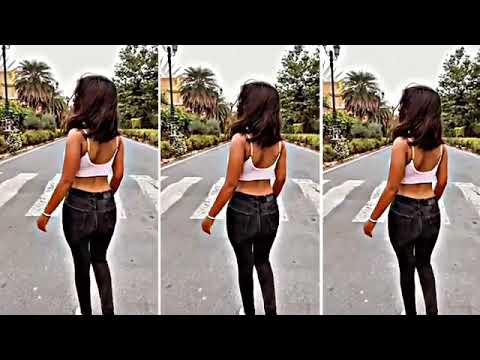The image is a triptych composed of three identical photos placed side by side, each framed by black borders at the top and bottom. The central focus in all three images is a young woman with tanned Caucasian skin and straight, shoulder-length brown hair being blown forward by the wind. She wears a white halter top and black skinny jeans, complemented by a white bracelet on her left hand. The woman stands in the center of a road marked by white lines, positioned such that we only see her back. Surrounding her in the distance is a tropical landscape featuring palm trees, other greenery, and some buildings, all under a gray sky. The scene appears to be captured in the middle of the day. Slight variations among the three images include differing views of her shoes, which are more visible in the rightmost photo compared to the center and left images.